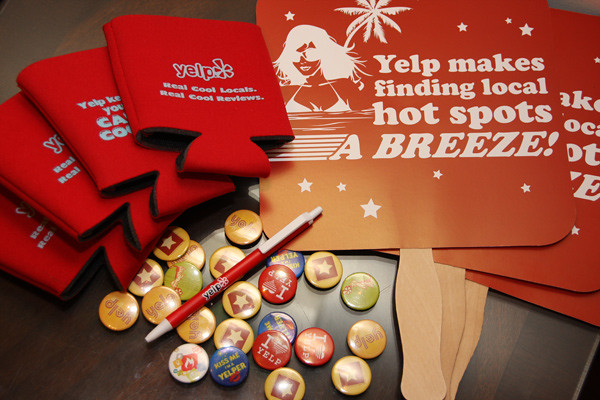The image depicts an array of Yelp merchandise artfully arranged on a dark wooden table. In the upper left corner, there are four red beer koozies fanned out, each featuring the Yelp logo and the phrase "Real cool locals, real cool reviews." Adjacent to the koozies are three paper fans resembling small signs, each mounted on a wooden stick with a design of a woman in sunglasses and a bikini, set against a palm tree backdrop, and emblazoned with the slogan "Yelp makes finding local hot spots a breeze." Spanning the bottom of the image is a colorful assortment of small buttons, some with messages like “I love Yelp” and “Kiss Me, I'm a Yelper,” each adorned with stars and other playful symbols. Among the buttons lies a red and white Yelp-branded pen, completing this vibrant display of promotional items.